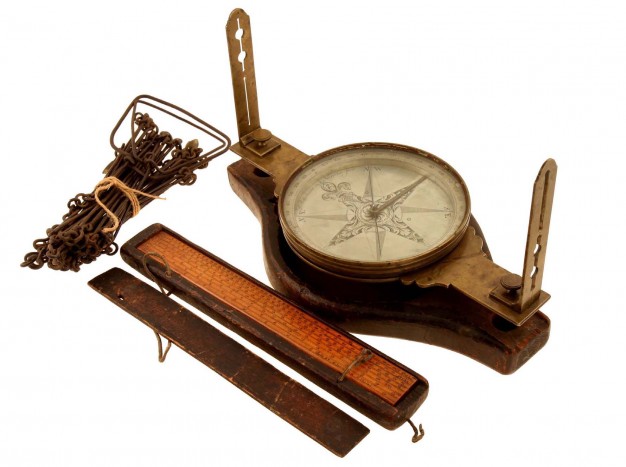The image showcases a collection of antique tools on an entirely white background. In the upper right-hand corner, there is an aged, rusty circular compass with a white back, light gray directional arrows, and hands, along with an eight-pointed star design in the center. The compass is partially encased in a bar that extends to the ends. In the upper left-hand corner, a bundle of old rusty metal stakes is neatly tied together with a piece of twine. Below, in the bottom left-hand corner, lies a set of wooden devices. One piece is a long, rectangular tool with a light wooden color in the middle and a brown border, possibly functioning as a ruler or edge smoother. A matching rectangular cover or additional piece lies adjacent, notable for its light orange top and dark brown wooden body, giving the impression of being part of a cohesive wooden toolset. The string or twine appearing in different sections of the image suggests potential hanging or binding purposes for these items.